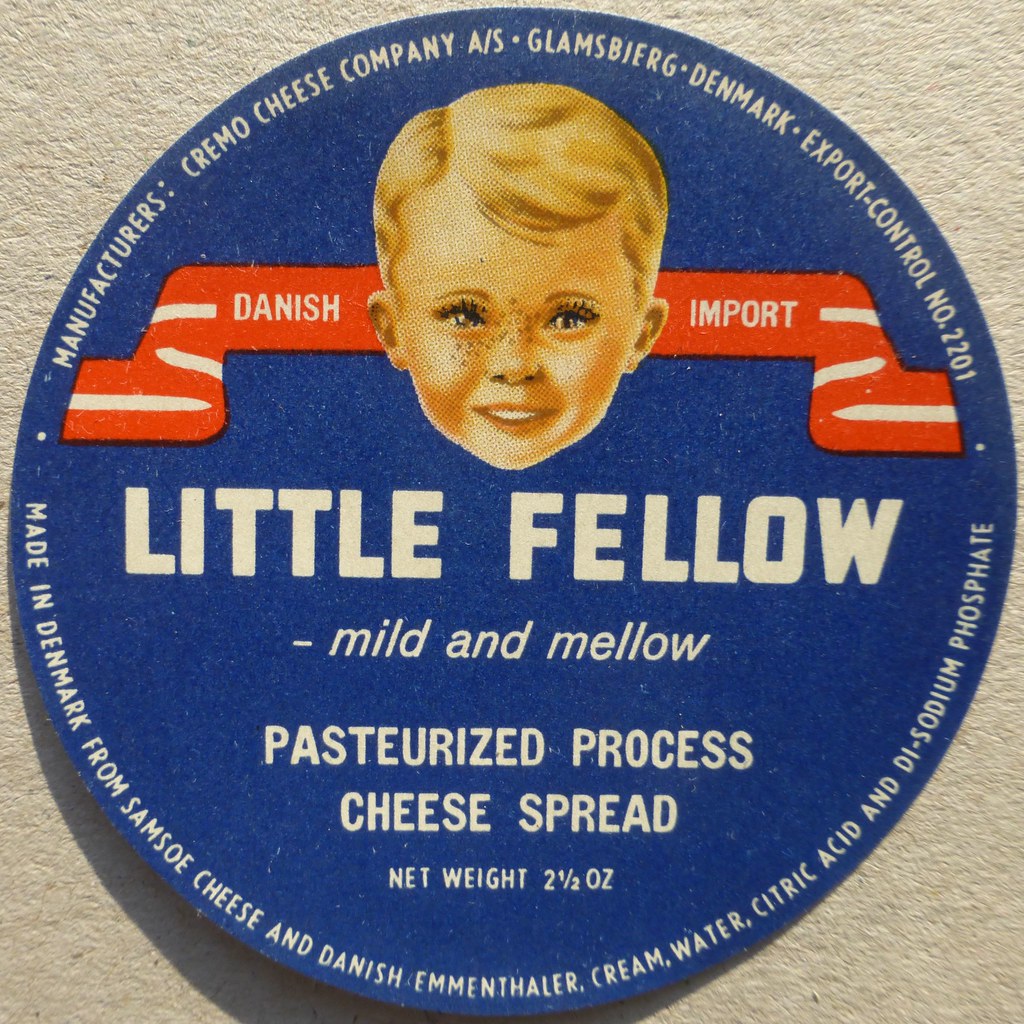The image presents a detailed, circular, dark blue label set against a light, textured stone surface, likely indoors. The label takes up nearly the entirety of the frame and is well-centered. At the top center of the label is a cartoon illustration of a blonde-haired, freckled, happy child with Caucasian skin and white eyes. The illustration is bordered by a red ribbon with white edges, stretching horizontally with "Danish" on the left and "Import" on the right, in white lettering. Above the child’s head, there’s small white text reading "Manufacturers, Cremo Cheese Company AS, Glamsburg, Denmark, Export Control Number 2201." Below the child's face, large white letters spell out "Littlefellow," followed by the phrases "Mild and Mellow" and "Pasteurized Processed Cheese Spread" in smaller fonts. The bottom section of the label lists "Net Weight 1 1/2 OZ" and "Made in Denmark from Samso Cheese, Danish Emmentaler, Cream, Water, Citric Acid, and Disodium Phosphate" in white text. The label appears to be affixed to the surface, possibly on a wall or a kitchen counter.